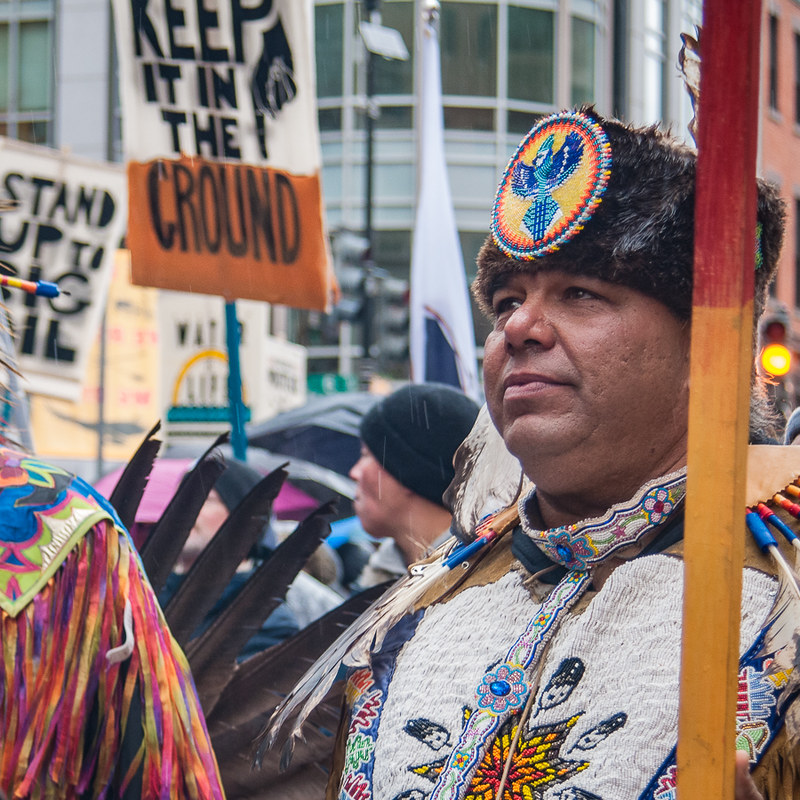The image captures a vibrant protest scene set in a city, focusing on a prominent Native American man dressed in traditional tribal clothing. He wears a distinctive fur hat adorned with a circular blue jay emblem, crafted from colorful beads or yarn. His multicolored outfit, embellished with intricate beadwork, feathers, and animal hide, features a unique white and brown pattern with floral motifs around the neck. To his left, another individual dons an eye-catching, rainbow-hued traditional garment accented with a striking plume of five large feathers. The background reveals a gathering of blurred protesters holding signs, with prominent slogans like "Keep it in the Ground" and "Stand up to Big Oil," advocating against oil drilling on indigenous lands. A mix of urban elements, including white and orange buildings and a car, completes the backdrop of this powerful demonstration.